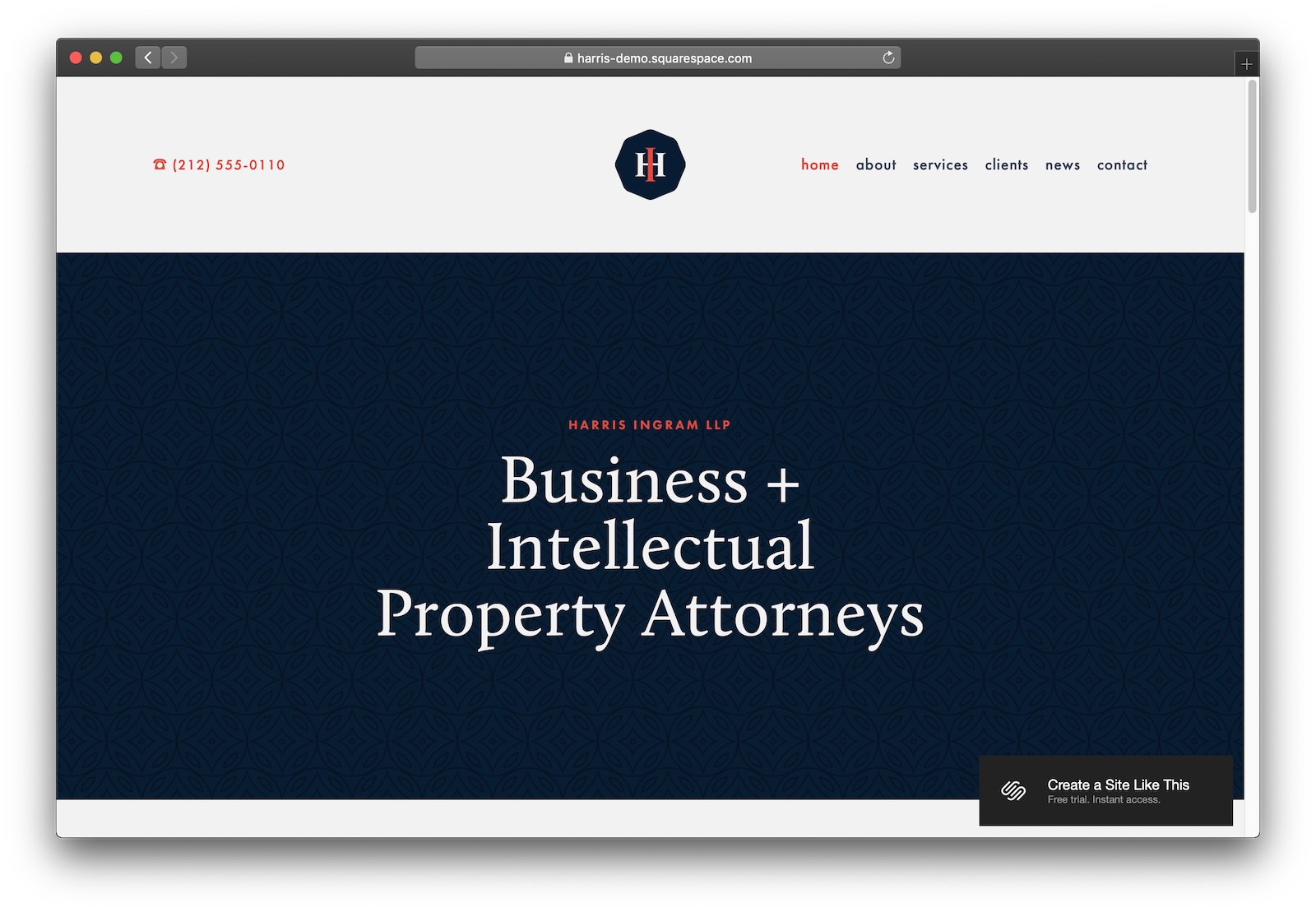The image depicts a webpage dedicated to site creation. In the top left corner, there is a prominently displayed contact number in orange: 212-555-0110, along with the country code. Centrally positioned on the page is the logo, while the top right section features navigation links including Home, About, Services, Clients, News, and Contacts. The page also includes additional text highlighting the firm's name, Harris Ingram LLP, and their specialization in business and intellectual property attorneys.